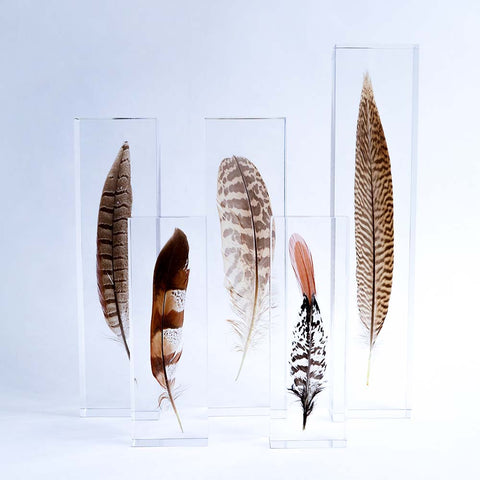The photograph showcases five large feathers displayed on a plain white background, each encased in clear glass cases. The feathers, likely from different species of birds, vary in size and exhibit a range of intricate patterns and colors. 

From left to right:
1. A predominantly brown feather adorned with approximately twelve horizontal black stripes.
2. A feather featuring five distinct sections: brown at the top, followed by white, a brown-reddish stripe, another white section, and culminating in a faint reddish-brown section before the stem.
3. An off-white feather decorated with grayish-brown striped patterns resembling a leopard print.
4. A white feather with black stripes and an orange-peach tip.
5. The longest feather, which is thin and brown, marked with darker brown stripes running its length.

All the feathers are positioned vertically, allowing the detailed patterns and colors to be clearly visible through the glass enclosures.